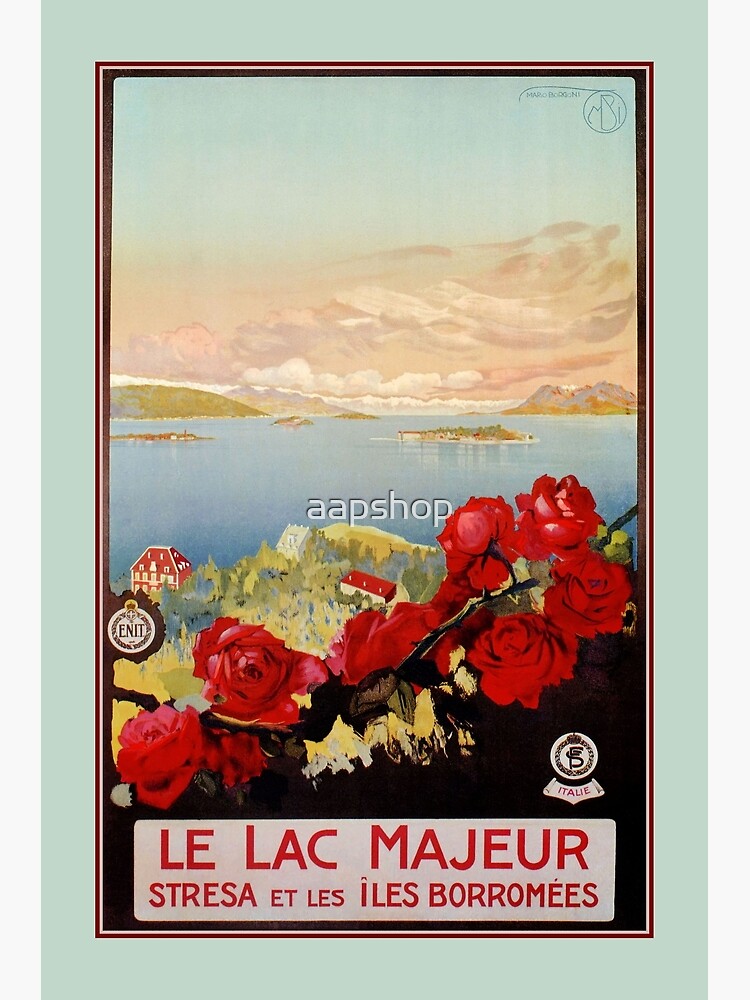This vintage travel poster, a digital reproduction by AAPSHOP, features a picturesque view of Lake Maggiore, inviting viewers to visit a scenic locale in Italy. In the foreground, vibrant red roses frame the scene, adding a burst of color. The perspective is from a hillside overlooking a quaint village nestled by the expansive lake. Two notable buildings with red roofs, one resembling a school and another shorter structure, add architectural interest to the densely forested area below. 

In the distance, mountains rise majestically, and a cluster of small islands can be seen dotting the lake's horizon. The sky exhibits hues of orange and yellow, suggesting a sunset ambiance. Promotional text at the bottom reads, "Le Lac Majeur" and "Stressa et Les Isles Borromées," hinting at the area's charm. Additional details include an emblem on the left corner, labeled "ENIT," and a symbol on the right, labeled "Italia." The entire scene is framed by a brown border with a pale blue edge, emphasizing its vintage allure.